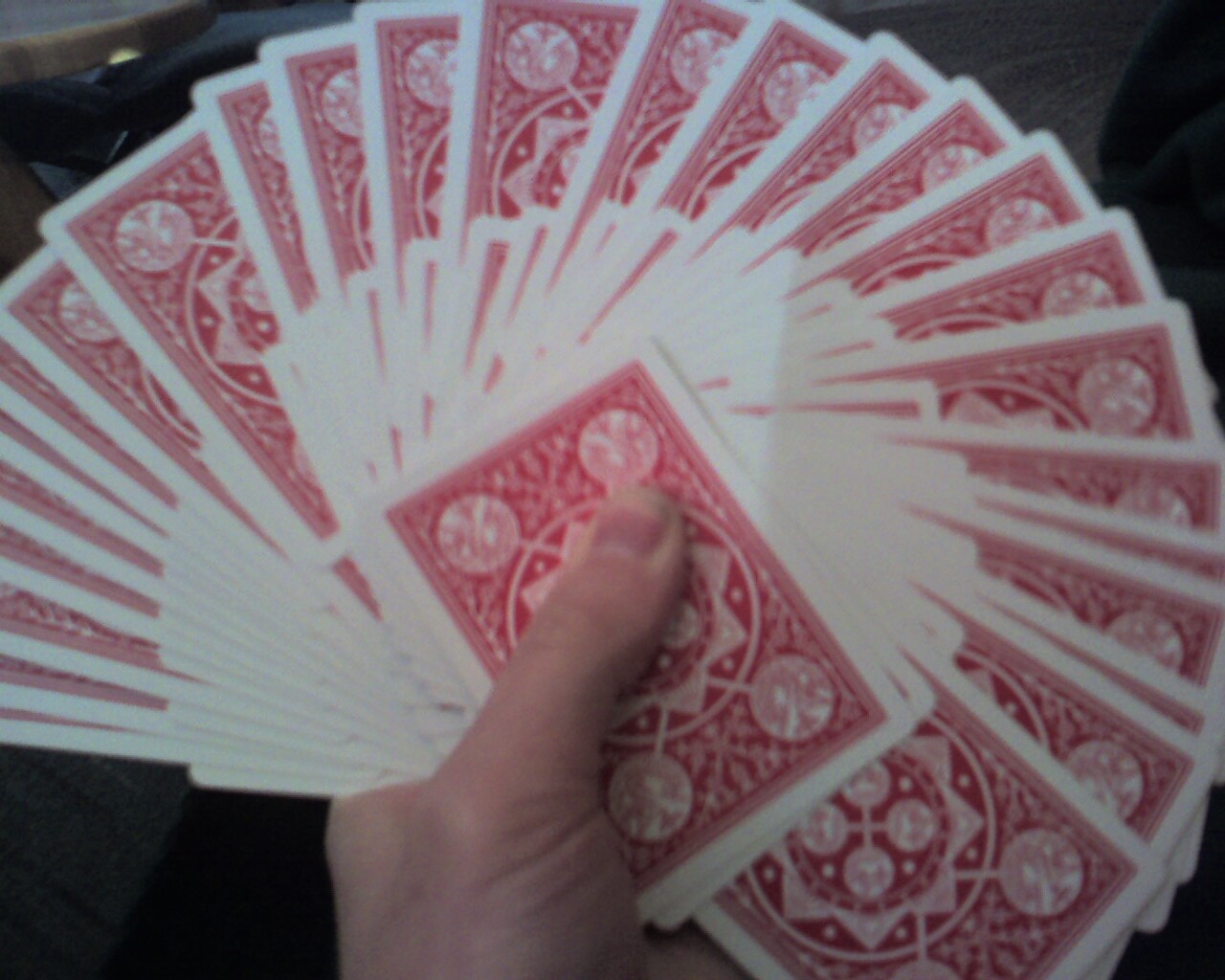A landscape-oriented photograph captures a fanned-out deck of cards held by a hand emerging from the bottom of the image. The thumb secures the cards, which are face down, revealing only their ornate backs. The intricate red and white design features a central flower surrounded by circles, with additional circles adorning each card's edge, all embellished with elaborate patterns. The cards, likely two full decks, span nearly the entire width of the image, occupying approximately 90% of the frame. The background appears pitch black, providing no discernible detail beyond the striking display of the cards.